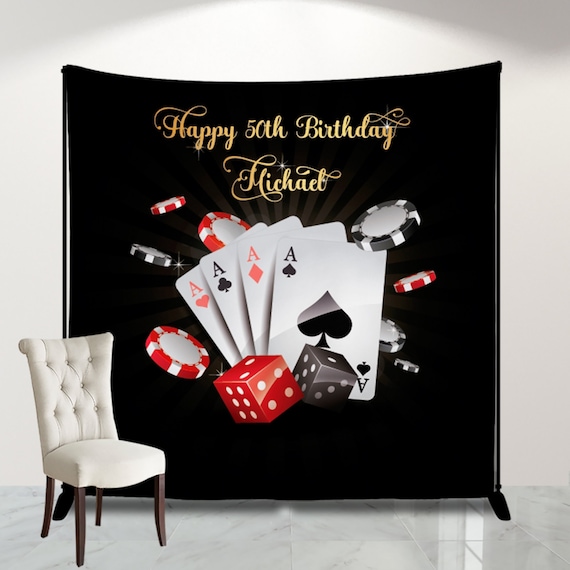The image portrays a digitally created scene with a large black banner hanging against a light-colored, possibly white wall. The banner prominently displays the text "Happy 50th Birthday Michael" in an elegant, gold cursive font. Centered on the banner are the four ace cards from a standard deck: ace of spades, ace of diamonds, ace of clubs, and ace of hearts. Surrounding these cards are red and black poker chips, seemingly spilling off to the sides. Additionally, a red die and a black die are positioned at an angle in front of the banner. Below this setup, the floor is a light gray, polished marble, reflecting light, and situated at the bottom left corner of the image is a white leather chair with a quilted back and brown legs. The overall lighting is subtle, casting soft streams of light that enhance the backdrop and floor's reflective quality.